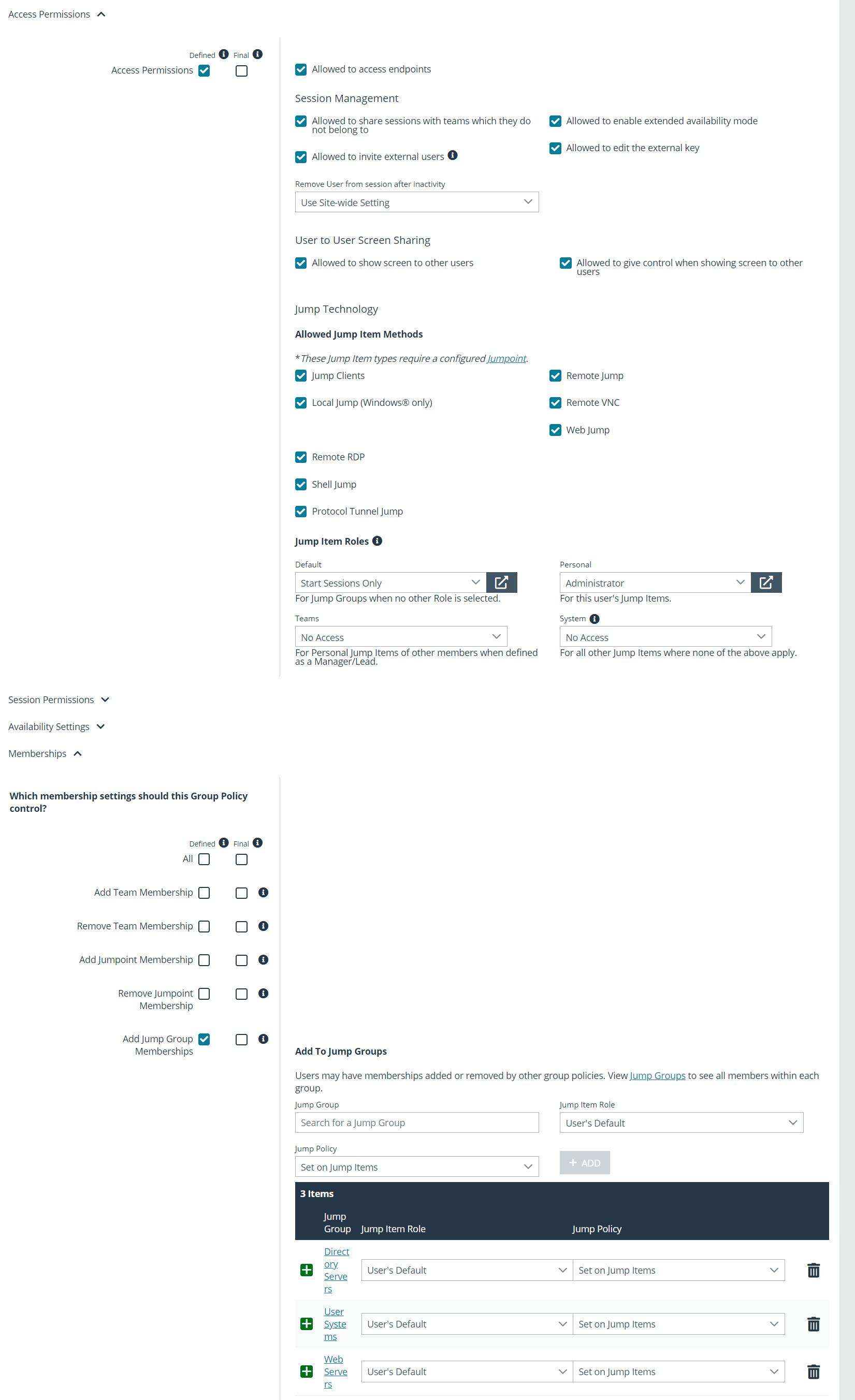This is an image of a cluttered and busy website, lacking a prominent title or clear headings. The website seems to be oriented towards managing account settings or permissions. 

On the right side of the image, there are several elements arranged in little boxes. One prominent feature is a blue checkbox with a white tick mark, indicating an active setting. Above an empty square, there are two round black circles. The text here, though difficult to read, includes phrases like "allowed to access" and "management." This right section is filled with checkboxes, most marked with blue ticks, and a noticeable black circle at the end of one of the lines.

Further down, a spacebar is visible with text below it that reads "use site web setting." Additional small, unreadable text seems to be indicating various permissions or options, such as "allowed to show screen to others," which is checked off, alongside another checkbox labeled "jump technology" which permits jumping, denoted by blue checkmarks. Below this, instructions like "jump something cheap" or "jump here" are mentioned. There are also two black boxes that resemble images of squares with nails through them.

Switching to the left section of the website, there are three distinct listings in black font at the top. This section is equally difficult to decipher, featuring bolded text in small writing. The left and right sides of this area contain vertical rows of boxes, and towards the middle, a larger solid black box with small images around it. At the bottom, green-colored boxes with bars for filling data and dropdown menus are present. 

Overall, the website is highly detailed but poorly organized, making it challenging to navigate or read the content effectively.